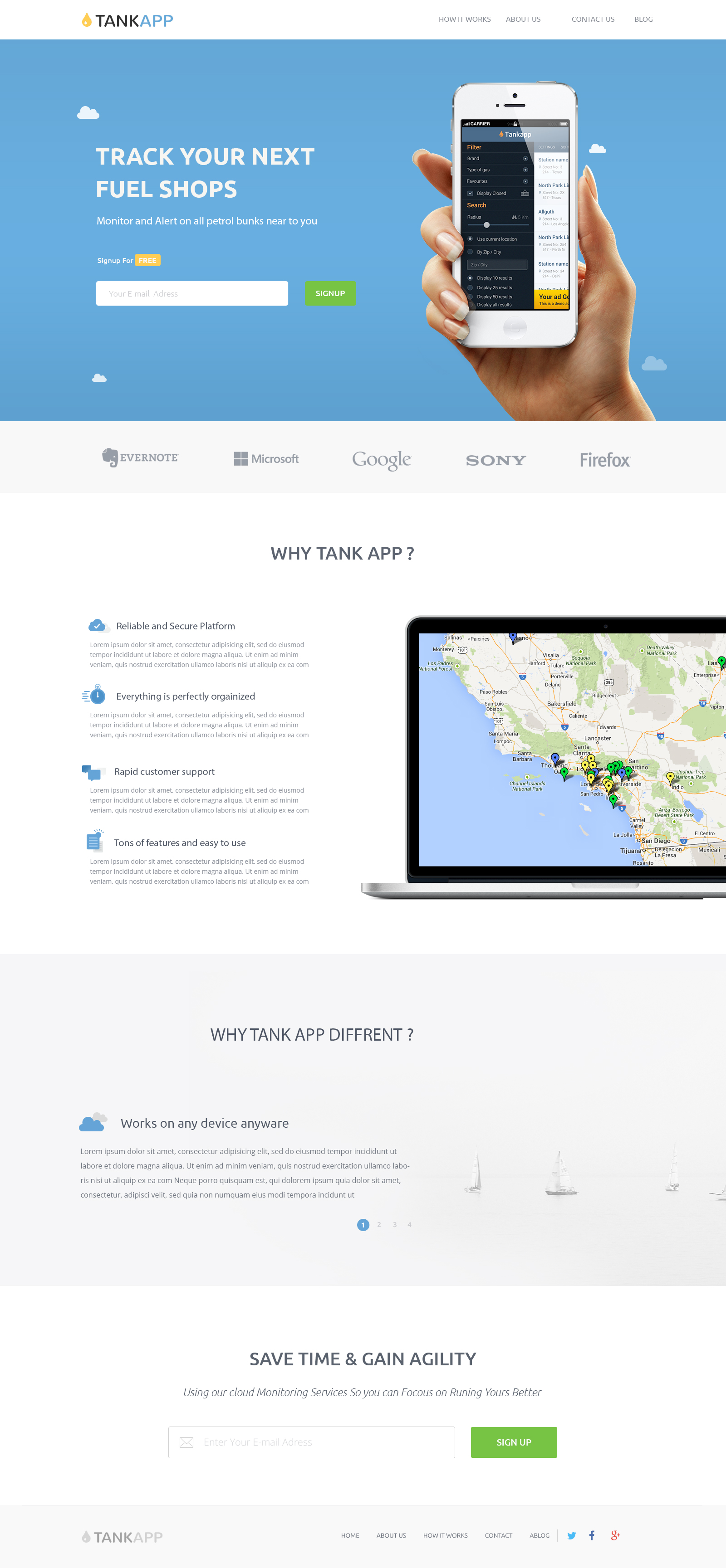A detailed screen capture from a website displaying the interface of the "TANK APP." At the top, a bold orange flame icon accompanies the name "TANK" written in black, all caps, followed by "APP" in blue, all caps. Below this header, there are small, unreadable subheader menus in black.

Dominating the page is a large blue rectangle. Inside this rectangle, white font reads "Track Your Next Fuel Shops." A white search box and a green box with white text are also present. A light-skinned woman’s hand, characterized by delicate nails, holds a white cell phone featuring a display with black, blue, white, and gold graphics. The blue rectangle's background includes subtle white clouds.

Beneath this, a sequence of familiar gray company icons is displayed: Evernote with an elephant icon, Microsoft's four squares, Google, Sony, and Firefox.

The text "Why Tank App?" appears against a white backdrop, followed by several sections, each containing a blue icon, a black header, and a brief paragraph of text—four sections in total. Adjacent to these sections is an image of a laptop with a black border and a silver body, showing a map with tan-green terrain, marked cities, multicolored icons, and blue and green water bodies.

A gray box with black text states "Why Tank App Different?" followed by a header section adorned with a blue cloud icon. The text "Work on Any Device Anywhere" appears in black, accompanied by a succinct paragraph. Further down, the phrase "Save Time and Gain Agility" is written in black, with additional explanatory text beneath it. 

At the page's bottom, there is a green box with white text, another mention of "TANK APP," and more black menu items. The final row consists of a blue icon, a gray icon, and a red icon, completing the visually detailed presentation of the website.